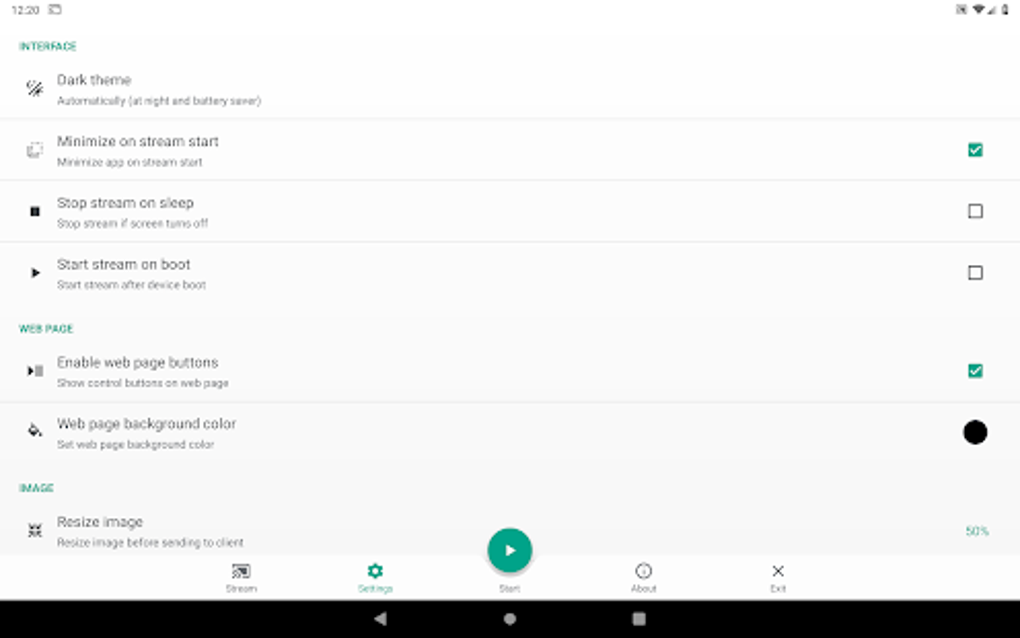The image depicts a user interface screenshot against a white or possibly grey background. At the top, black text reads "1220", followed by an Instagram photo icon. On the far left side, there is a black box displaying full Wi-Fi signal, low cell service, and a nearly depleted battery indicator.

Along the left-hand side, the interface displays a menu with the following options:
- Dark Theme
- Minimize on Start
- Stop Stream on Sleep
- Start Stream on Boot
- Enable Webpage Buttons
- Enable Webpage Background Color
- Resize Image

Each menu option has accompanying text that is too small to read clearly due to the size and resolution of the screenshot.

Towards the bottom center of the image, there is a section labeled "Stream Setting" with a green button featuring a white arrow pointing to the right, likely labeled "Start". Below this are two more options: "About" and "Exit".

At the very bottom, a black bar runs across the width of the image. In the center of this bar, there is a circle; to its left is a left-pointing arrow, and to its right is a square icon.